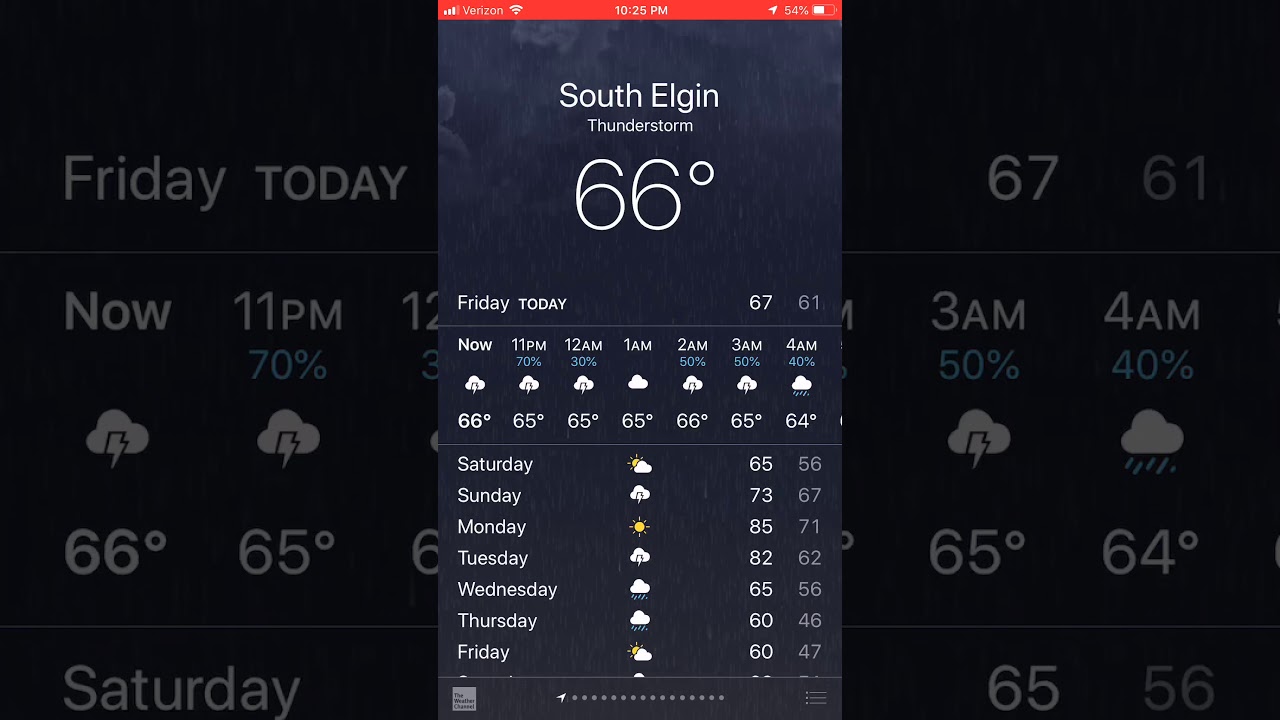The landscape-oriented screenshot captures the display of a smartphone screen placed at its center. The smartphone's screen exhibits a red bar at the top, prominently displaying the time as 10:25 p.m. Lowering from the red bar, the background shifts to a dark gray hue. In the upper-middle part of the screen, white text denotes the current location as South Elgin, the weather condition as a thunderstorm, and the temperature as 66 degrees. Beneath this, a detailed table lists the days of the week, weather conditions for each day, and corresponding temperatures. Accompanying the weather descriptions are various icons symbolizing different weather conditions, including a cloud, the sun peeking from behind a cloud, lightning striking from a cloud, a solitary sun, and rain beneath clouds.